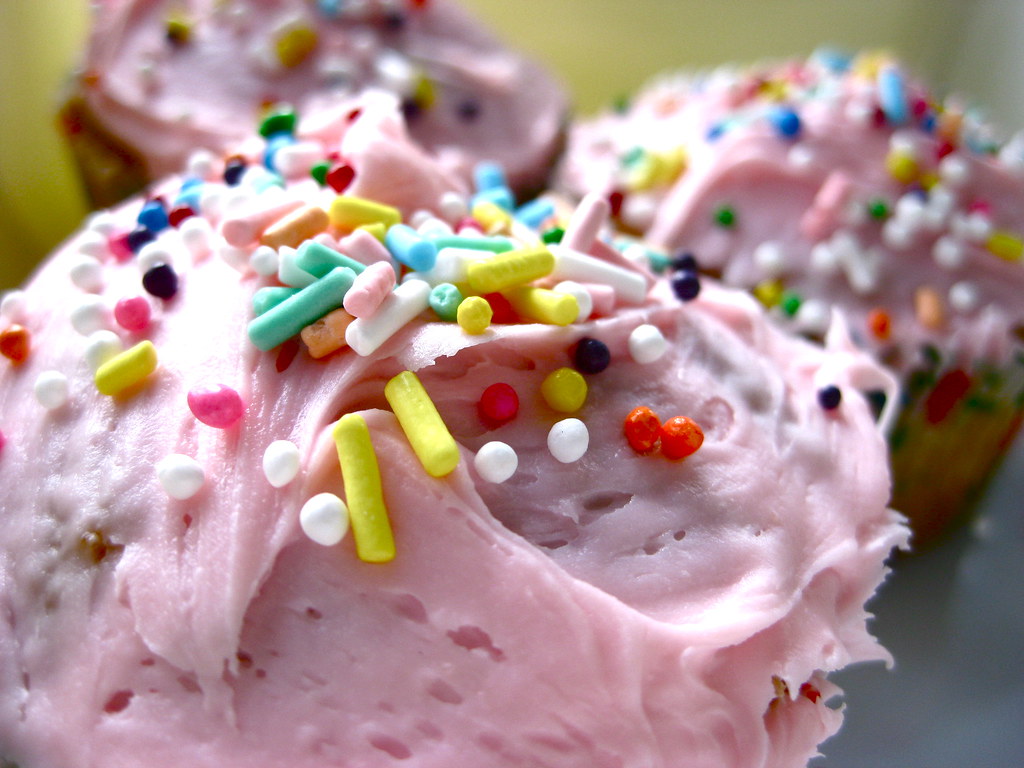This close-up image features three cupcakes adorned with light pink icing and a variety of colorful sprinkles. The foremost cupcake is in sharp focus, showcasing its detailed decoration, while the two cupcakes behind it are slightly blurred. The sprinkles vary in color, including yellow, white, green, blue, red, black, orange, teal, and pink, and come in both cylindrical and spherical shapes. The cupcakes are set on a shiny, gray surface, likely a plate or countertop, with a yellow wall providing a soft background contrast. Notably, the cupcakes themselves have a golden-brown hue typical of freshly baked goods. This image captures the intricate details of the cupcakes, emphasizing their vibrant sprinkles and inviting appearance.